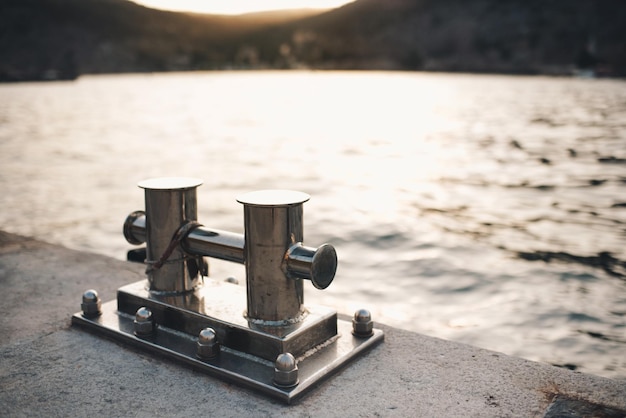The image depicts a stainless steel cleat securely fastened to a concrete dock with multiple bolts, ensuring a firm attachment for securing a boat. The cleat, used for tying boats to the dock with ropes, is the focal point of the image and is sharply in focus, standing out against the grayish-silver tones of the concrete. Beyond the cleat, the background is slightly blurred, showcasing a tranquil lake with a faint shoreline of trees and possibly a hilly or mountainous landscape. The entire scene evokes a scene of a mooring spot at a lake or harbor, with calm waters and subtle natural colors adding to the serene atmosphere.